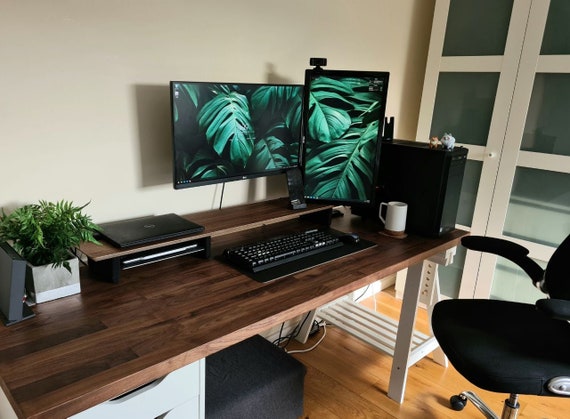This photograph showcases a meticulously arranged home office set against a backdrop of a light gray wall. The focal point is a desk featuring a large rectangular dark wood top with white legs, positioned against the wall. On the right side of the image, a black rolling computer chair is turned sideways, revealing a warm golden-yellow wooden floor beneath.

On top of the desk, a black keyboard rests centrally on a black mat. To the right of the keyboard, there is a white tea mug. Behind the mug, a black computer monitor stands out, next to which two additional screens are visible. One monitor is set up horizontally, while the other is positioned vertically with a camera mounted on top. Both displays exhibit a vivid plant-based design dominated by green leaves.

To the left of the monitors, a Wi-Fi router and a small house plant add a touch of greenery and connectivity to the workspace. A laptop is also present on a smaller shelf toward the back of the desk.

Underneath the desk, there are two storage bins—one black and one white—providing additional organization. In the background, a white cabinet with glass-paneled doors offers further storage solutions, enhancing the functionality of this serene and stylish home office.